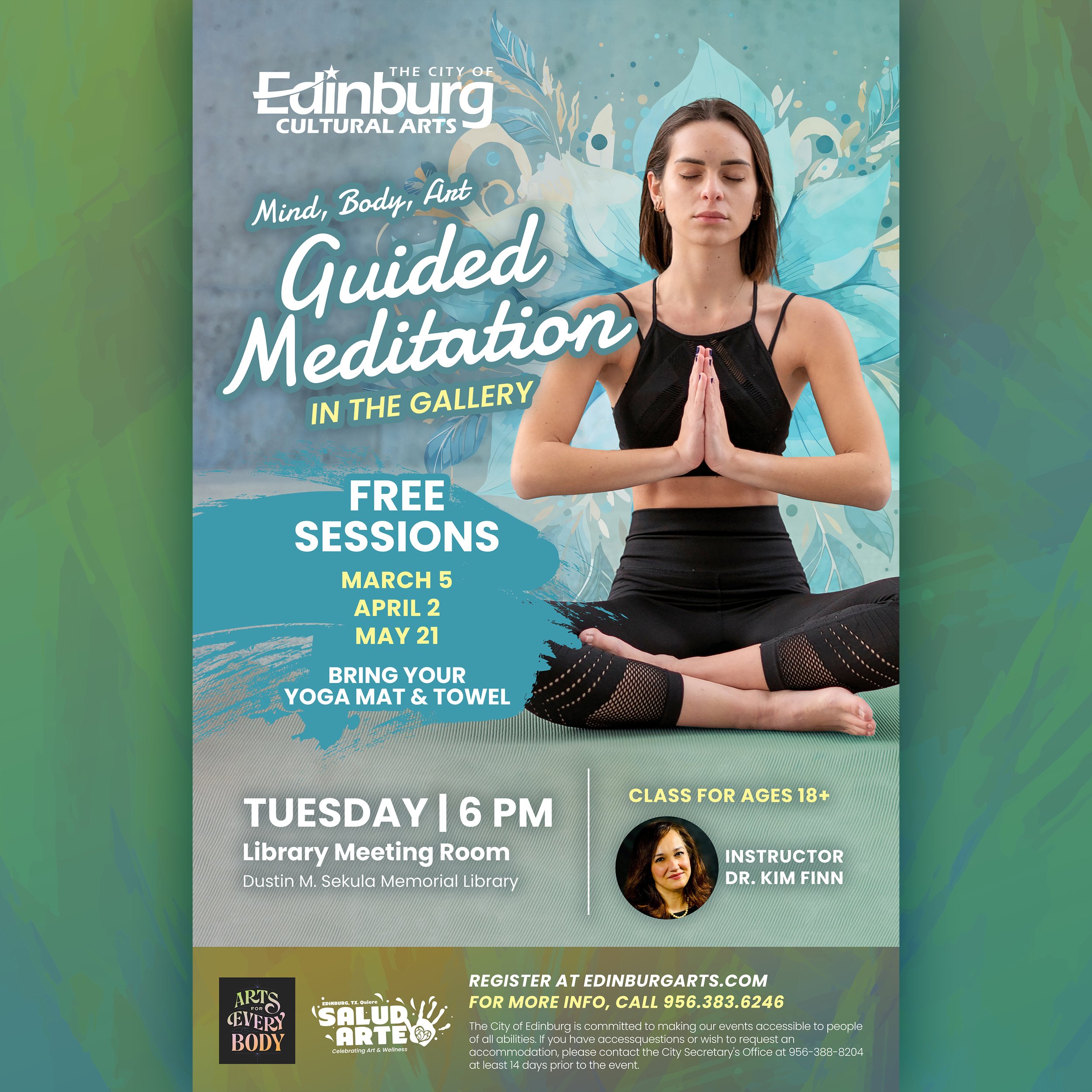The image is a square-shaped advertisement flyer with a greenish-blue pastel background. In the center, there is an upright rectangular photograph of a young Caucasian woman with short brunette hair flowing down her back. She is sitting cross-legged in a yoga pose, wearing a black crop top and black leggings. Her hands are together in a praying symbol in front of her chest, and her eyes are closed, evoking a sense of calm and focus. Behind her, there is a light blue lotus flower design, adding to the serene atmosphere of the flyer.

The text on the flyer includes the following details:
- At the top, it says "The City of Edinburgh Cultural Arts" in white.
- Below that, in a script font, it reads "Mind, Body, Art: Guided Meditation."
- In bold, all caps, it states, "IN THE GALLERY."
- Further down, it informs about "Free Sessions" on March 5th, April 2nd, and May 21st.
- Attendees are asked to "Bring your yoga mat and towel."
- The sessions are held on Tuesdays at 6 p.m. in the Library Meeting Room of the Dustin M. Circula Memorial Library.
- The classes are for ages 18 and above.
- The instructor is Dr. Kim Finn.
- To register, visit edinburgharts.com or call 956-383-6246 for more information.
- Additional information at the bottom mentions the city’s commitment to accessibility, urging individuals with access questions or the need for accommodations to contact the city secretary's office at 956-388-8204 at least 14 days prior to the event.

The flyer also includes logos for "Arts for Everybody" and "Salud Art," enhancing its community-centric appeal.